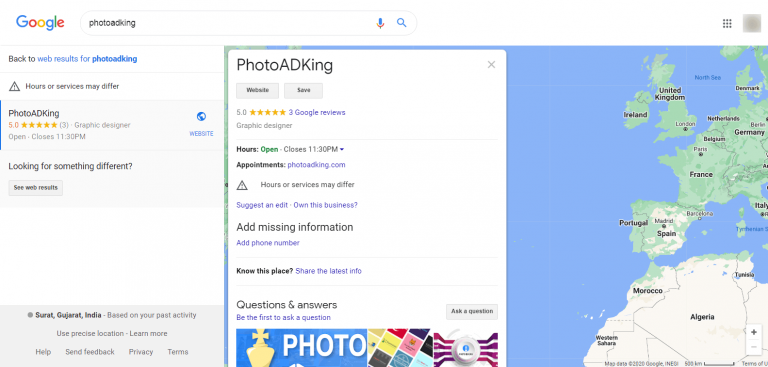The image displays a Google search result page. In the top-left corner, the Google logo is prominently featured with its familiar colors: blue, red, yellow, blue, and red. Beneath the logo, black text reads "Photo AD King." Below, the search results include a listing for "Photo AD King" with five stars based on three ratings. The business is labeled as a graphic designer, and it notes that it closes at 11:30 PM.

On the right side of the page, the section showcases appointment options for Photo AD King, with a link to "photoadking.com." Below this, options appear to add missing information and to access a "Know this place?" section for questions and answers.

The right-hand panel also displays a map featuring various geographic locations. Although the exact location isn't clear, browsing history suggests users have searched from Surat, Gujarat, India, as well as countries like Ireland, the United Kingdom, the Netherlands, Germany, France, Spain, Portugal, Italy, Algeria, and the North Sea region. Various textual elements and additional data are visible throughout the page.